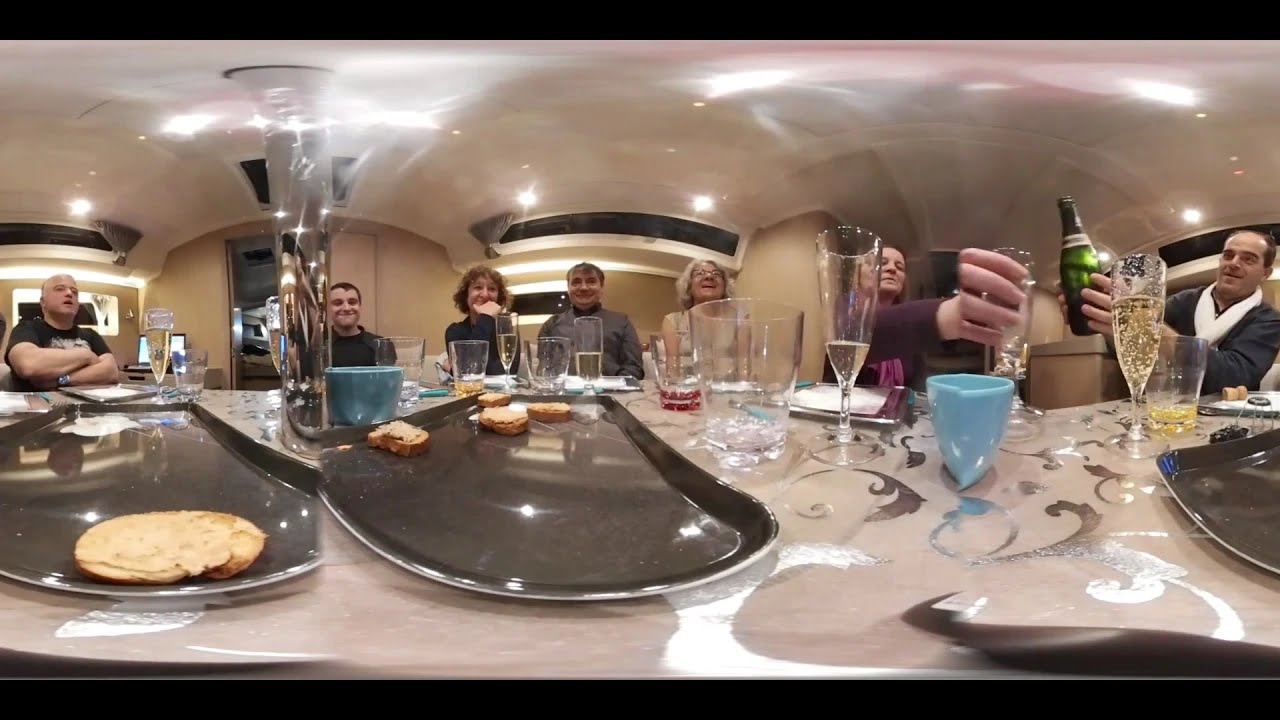This horizontal rectangular image, framed with black borders at the top and bottom, captures a lively dinner scene shot with an unusual lens that creates a curved and distorted effect. The distortion makes the objects on the table appear exaggeratedly large compared to the people behind them. The table, possibly a bar, is strewn with plates, some largely emptied of food, and various drink glasses. In the foreground, a glass seemingly filled with silverware is visible among the disheveled dining setting.

Behind the table, eight individuals are arranged, all facing the viewer. The focal point includes three people directly in front, with one appearing to eat. To the right, a man distinguished by a white scarf is pouring champagne from a bottle, his actions rendered intimate as only his hands are primarily visible. The scene exudes a cheerful and warm atmosphere with people smiling, further highlighted by the interaction of the man pouring drinks for another guest amidst festive trays of cookies or pastries.